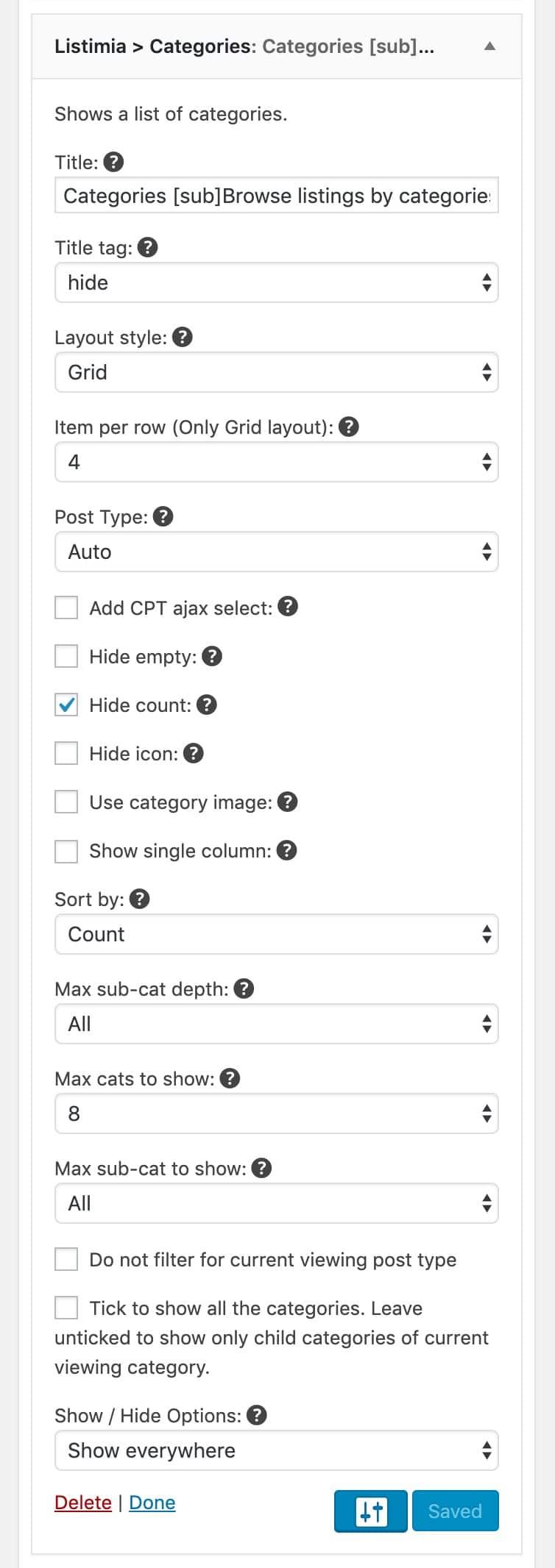This image displays a screenshot from a cell phone screen showcasing the settings interface of an app or software for listing categories. The interface prominently features multiple configurable options and detailed settings. At the top, the title "Categories (Sub)" is noted, accompanied by a brief description: "Browse listings by categories." 

Below the title section, various field labels such as "Title Tag," "Hide," "Layout Style," "Items per Row," and "Post Type" are present. The "Layout Style" is set to "Grid," with "Items per Row" specified as "4," and the "Post Type" is labeled "Auto."

In the mid-section, six clickable option boxes are aligned vertically. The third box, labeled "Hide Count," has been selected, while other options like "Add CPT," "Hide Empty," "Hide Icon," "Use Category Image," and "Show Single Column" remain unselected. Each of these options includes a white question mark within a black circle, suggesting the availability of additional help or information.

Further down, the screen displays more settings, including "Sort by" (with the option set to "Count"), "Max Sub Cat Depth" (set to "All"), "Max Cats Show" (set to "8"), and "Max Sub Cat to Show" (set to "All"). Each of these settings is also accompanied by a white question mark in a black circle, indicating the potential for more detailed explanations or guides.